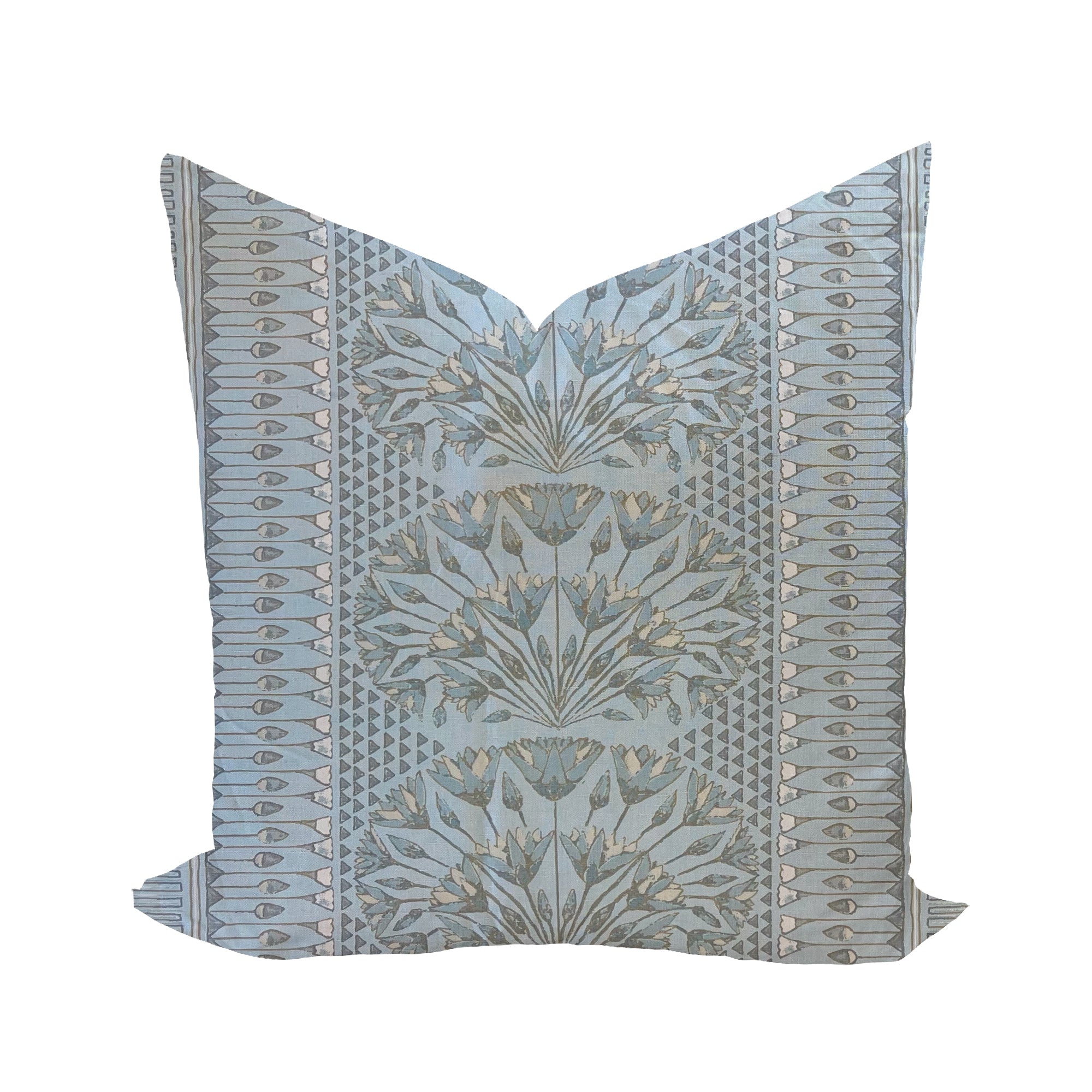This is an image of a decorative throw pillow positioned upright against a pure white background, giving no indication of its surroundings. The pillow, which is square in shape with a distinctive V-shaped indent across the top, appears to be purposefully styled for aesthetic presentation. The pillow's design features a central motif resembling three rows of floral patterns that radiate from a common center, forming rounded arches. These floral embellishments are predominantly in light blue and white tones. Flanking the central design are triangular patterns, and the outer edges display additional gray and white floral motifs pointing inward. The pillow is predominantly a bluish-gray color with various blue hues and white accents adding to its intricate, artistic appeal.